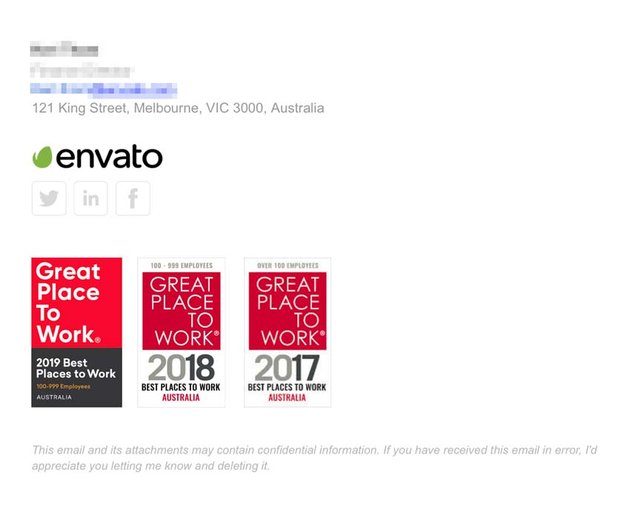The promotional image for the brand Envato elegantly presents its corporate details and accolades. The brand name "envato" is styled in lowercase, black font situated prominently on the image. To the left of the name, there's a distinctive, cute green circular icon with a tail-like extension.

Positioned above "envato," the address reads: 121 King Street, Melbourne, Vic 3000, Australia. Some text above the address is blurred, adding a subtle touch of mystery to the header.

Directly below the brand name, icons for Twitter, Instagram, and Facebook are displayed in individual gray square boxes, signifying Envato's social media presence.

The image also highlights Envato's commendable workplace achievements. Three colorful blocks, conveying their 'Great Place to Work' accolades, are displayed. 

1. The first block, divided into red and black halves, announces that Envato was voted a great place to work in 2019 by 100 to 99 employees. 
2. The second block, in red and white halves, celebrates the 2018 best place to work award in Australia.
3. The third block, also in red and white halves, honors the 2017 best place to work recognition in Australia. 

Each award block features the "Great Place to Work" text in white lettered red portions, with the respective years indicated in the white sections at the bottom. The year digits are color-coded with black for '18' and '17', and gray for '20' in '2017.'

A subtle disclaimer is also included, indicating that the email and its attachments may contain confidential information and advising proper action in case of erroneous receipt, suggesting that this image might originate from an email.

The background of the image is predominantly white, creating a clean and modern aesthetic.